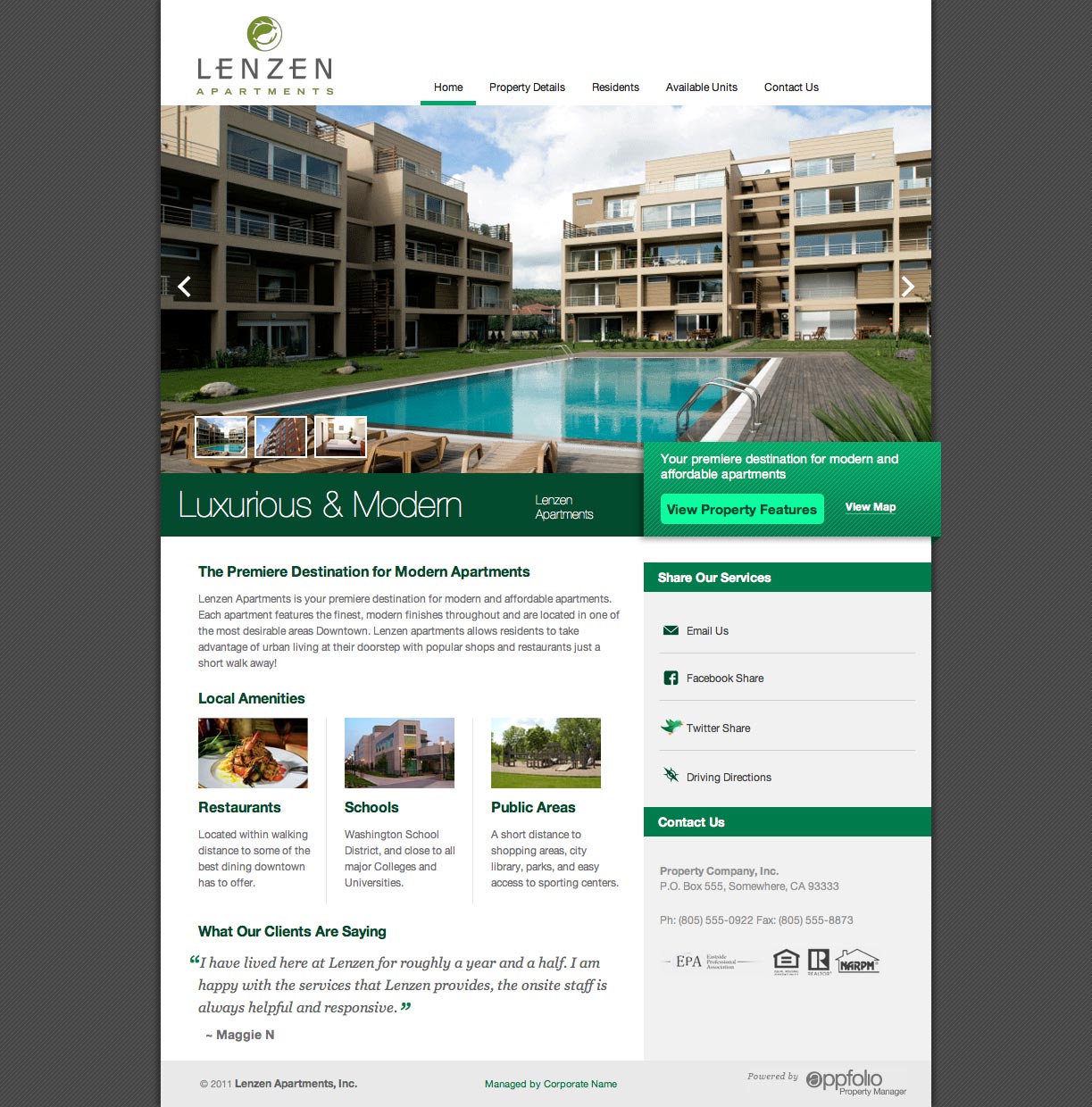**Lenzen Apartments Homepage Overview**

Welcome to Lenzen Apartments, an epitome of luxurious and modern living, located in one of the most desirable areas of downtown. The homepage features an elegant layout with top navigation links to Home, Property Details, Residence, Available Units, and Contact Us.

The main image showcases a stunning view of two sleek, modern apartment buildings, each rising four to five stories high, surrounding a sparkling pool. This visual immediately conveys the upscale and serene ambiance of the complex. Additional images of the property are available but not visible from the current view.

The accompanying text highlights Lenzen Apartments as the premier destination for modern living, emphasizing the luxurious finishes and desirable downtown location. The detailed description promises an unparalleled living experience with access to local amenities such as restaurants, schools, and public areas, each accessible through clickable links for more information.

A testimonial section features a glowing review from resident Maggie N., who has lived at Lenzen for a year and a half and praises the helpful and responsive online staff.

The right sidebar includes social media links to Facebook and Twitter, a map with a link to directions, and a 'Contact Us' section located at the bottom right of the page, ensuring visitors can easily connect with the leasing office.

The page design is predominantly white, complemented by tasteful green elements, contributing to the clean, modern aesthetic.